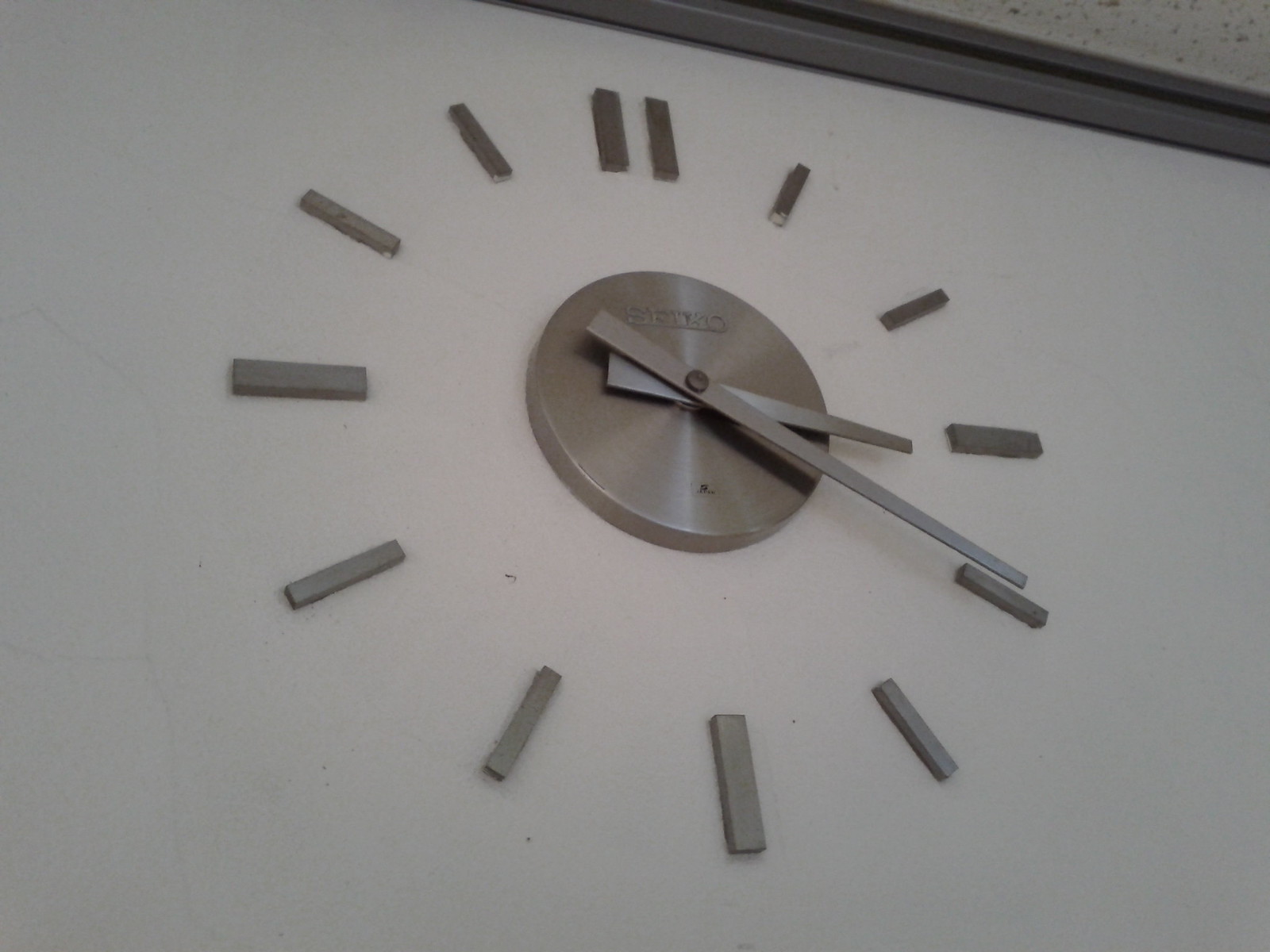This image showcases a close-up of a modern, simplistic wall clock mounted on a white background. The clock features no border, giving it a minimalist design. The face of the clock is defined by gray, silver dashes representing the hours from 1 to 12, instead of numerical digits. At the center of the clock, there is a stainless steel circle with the brand name "Seiko" stamped above the clock hands. Both the hour and minute hands are also made of stainless steel. The current time displayed is approximately 3:19 or 3:20. Shadows of the hands are visible on the clock face, adding a subtle depth to the image. The top right corner of the image reveals a gray trim separating the wall from what appears to be white ceiling tiles.